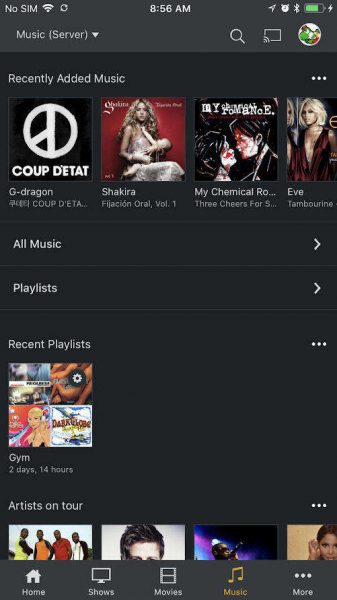The image is a screenshot from a mobile music application. At the very top, there is a light gray border displaying the status bar with the current time, battery icon, Bluetooth symbol, and an alarm icon indicating an active alarm. It also shows that there is no SIM card in the device.

Beneath this, there is a header titled "Music Server" with a dropdown icon to its right. In the top right corner of the screen, there are icons for search, casting to another device or screen, and the user profile avatar.

Following the header is a section labeled "Recently Added Music" featuring album cover art. The albums displayed are from artists including G-Dragon, Shakira, My Chemical Romance, and Eve.

Below this section are tabs for "All Music" and "Playlist." Further down, there is a section titled "Recent Playlist," showcasing a collage of four album covers, representing the contents of the playlist.

At the very bottom of the screen is a partially visible section labeled "Artists on Tour," with the artists' names partially cut off. The footer of the app displays navigation tabs for Home, Shows, Movies, Music, and More.